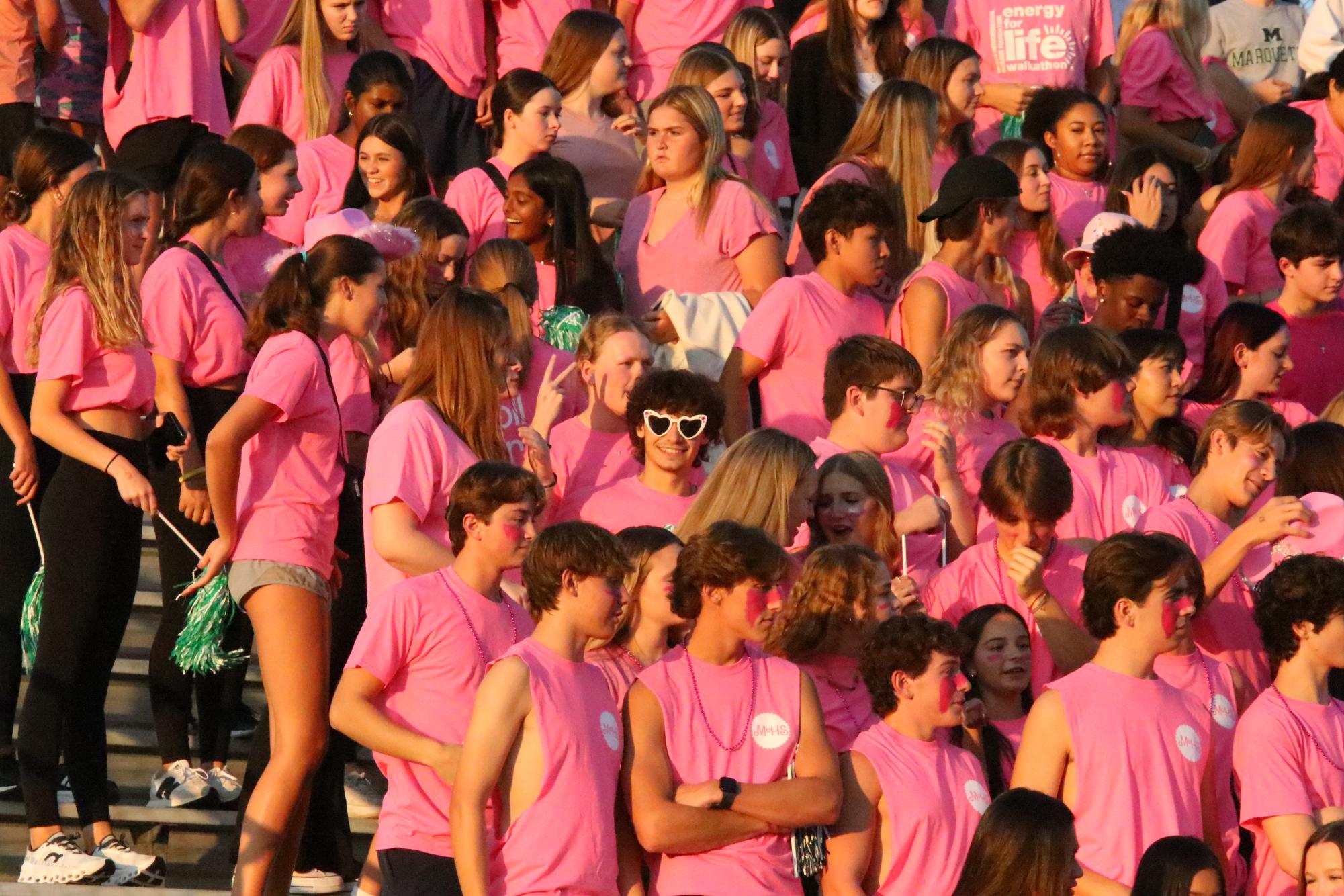The photograph showcases a lively crowd of predominantly teenagers and young adults, both males and females, gathered in bleachers. Most are dressed uniformly in pink shirts, some short-sleeved and others sleeveless, with a few exceptions where individuals wear different colored shirts, including a noticeable Marquette shirt in the upper right corner. The pink shirts often feature a white logo on the chest, though not everyone has this detail. The crowd, primarily composed of Caucasian teens with some diversity, includes a few black individuals. Many of the girls are clad in black leggings and white tennis shoes, while some opt for jean shorts. Accessories like sunglasses with heart-shaped lenses and green tassels add extra flair to the scene. Faces painted red are visible in the front row and middle sections, enhancing the energetic atmosphere which seems fitting for a sporting event or a large school gathering.